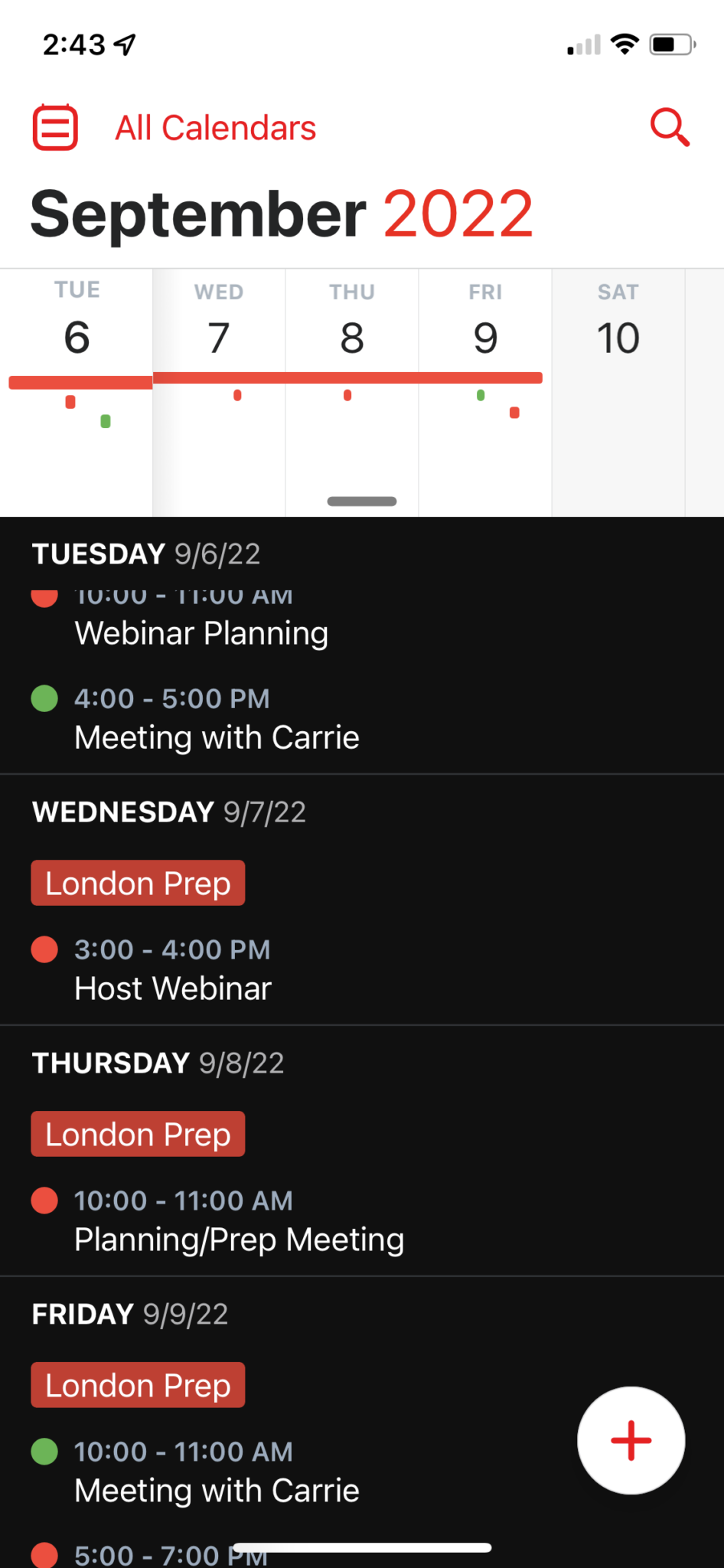The image displays a smartphone screen featuring a detailed calendar app interface. At the top of the screen, the time reads "2:43," with a small error icon positioned to its right. There is a series of connectivity bars indicating the signal strength: one black bar is lit up while the remaining three are gray. This is followed by a satellite icon and a battery indicator showing approximately 50% charge.

Beneath the status indicators is a search bar with a magnifying glass icon on the right and a small square icon with two lines on the left. The main part of the screen is titled "All Calendars," and just below this, it reads "September 2022" in larger text. The calendar layout spans across five rows, each representing a single week, with columns for each day from Tuesday to Saturday. The days are populated with dates, starting with "6" under Tuesday and progressing sequentially to "10" under Saturday.

Events are highlighted with red lines and dots, as well as green dots on certain dates. A notable detail is a prominent black box under Tuesday, specifying "Tuesday 9-6-22" with scheduled events listed such as "Webinar Planning" and "Meeting with Carrie," each accompanied by their corresponding times. Similarly, "Wednesday 9-7-22" lists "London Prep" from 3-4pm and "Host Webinar," followed by events on Thursday.

Towards the bottom right of the screen, there is a large white circle with a red cross inside, resembling an add or create button. Finally, a white line extends across the bottom edge of the screen, possibly indicating the navigation bar.